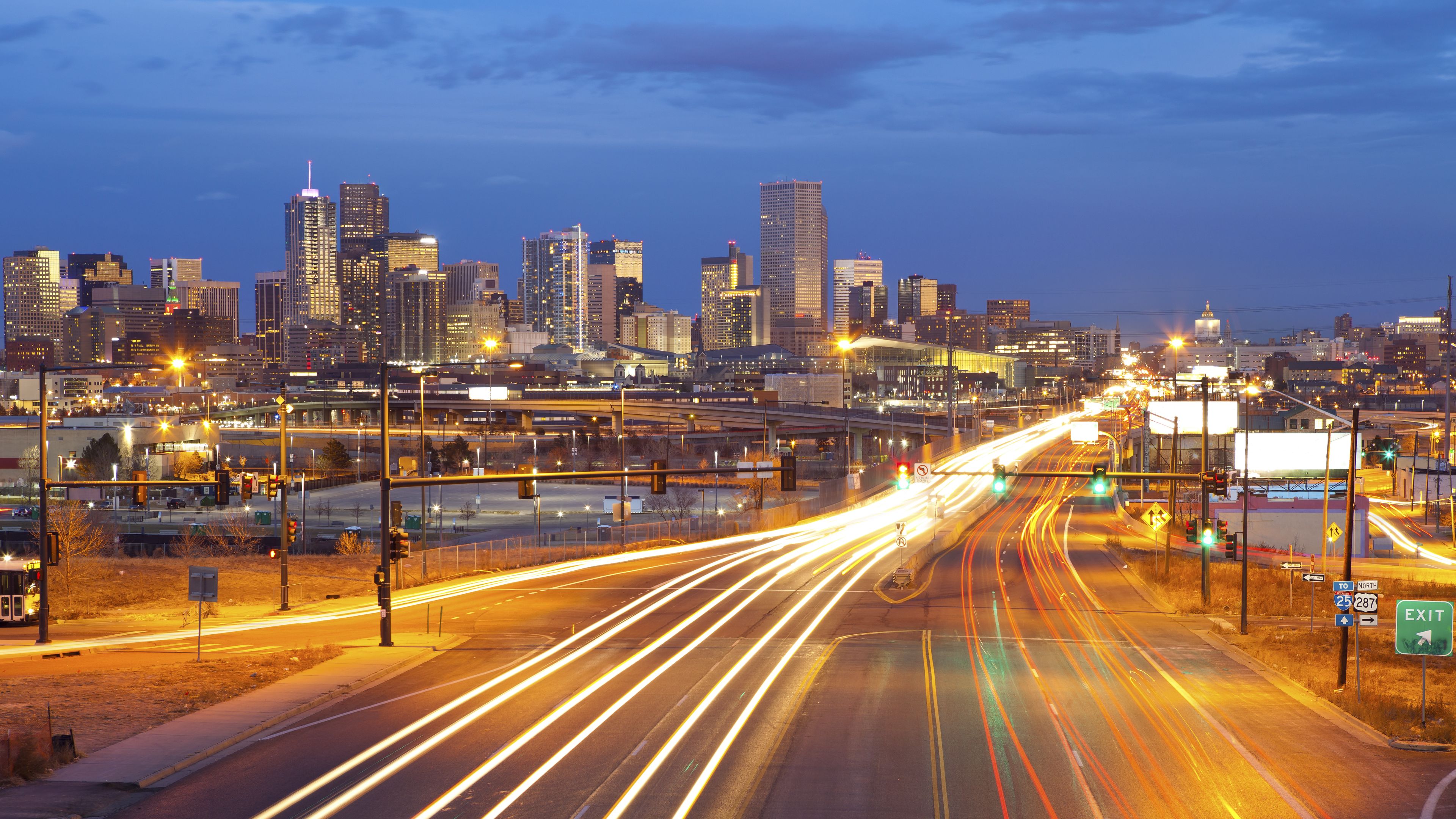This image captures a bustling nighttime city scene centered around a brightly illuminated freeway. The highway, comprised of two lanes in each direction, dominates the middle of the photograph, curving around a dense cityscape and eventually fading into the distance. Bright light trails—amber on the left, likely from streetlights, and red on the right, from vehicle brake lights—create dynamic lines across the road that suggest heavy, fast-moving traffic. Despite this, no individual cars or people are visible.

To the bottom right, an exit sign and additional directional signs point towards various paths. The city skyline looms towards the left, featuring an array of towering high-rises, one of which prominently features a white point at its summit. The high-rises are alive with countless lit windows, adding to the vibrant ambiance of the scene.

The sky is a deepening twilight blue, dotted with clouds but devoid of the sun, indicating that nighttime is setting in. The scene is dry, with no signs of rain, suggesting it was a pleasant evening. The image not only highlights the urban architecture but also captures the energy and movement of the city as it transitions into night.